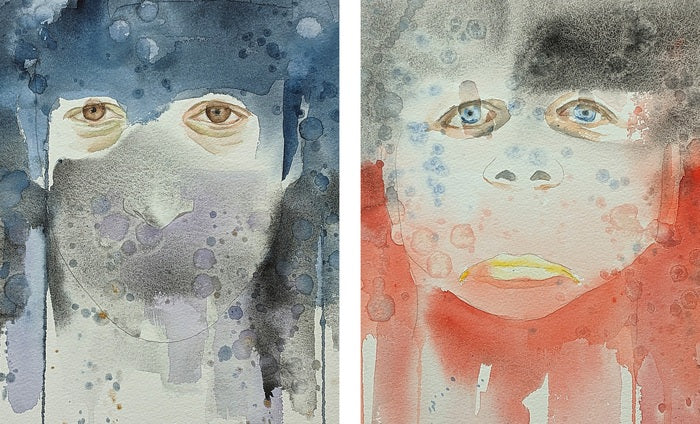This image showcases two striking watercolor paintings side by side, both primarily focused on expressive faces rendered with a mix of vivid and subdued hues. The left painting features a face with pale white skin, partially obscured by blue watercolor resembling a mask or headdress, and overlaid with black detailing that highlights tired, brown eyes with noticeable bags underneath. The face lacks a visible mouth and has a downturned, beak-like nose. Streaks of blue extend from the top, resembling hair, with subtle purple streaks and splatters adding depth and texture.

In contrast, the right painting depicts a face adorned with a vibrant red area around the head, suggestive of a helmet, transitioning to black at the top where the hair would be. This face has striking blue eyes accented with rings around them and features a distinct upturned nose. Golden lips stand out prominently against the surrounding colors, adding a touch of warmth to the otherwise cool-toned portrait. Splashes of blue are lightly scattered across the face, and the red coloration appears to drip down from the middle, creating a visually dynamic effect.